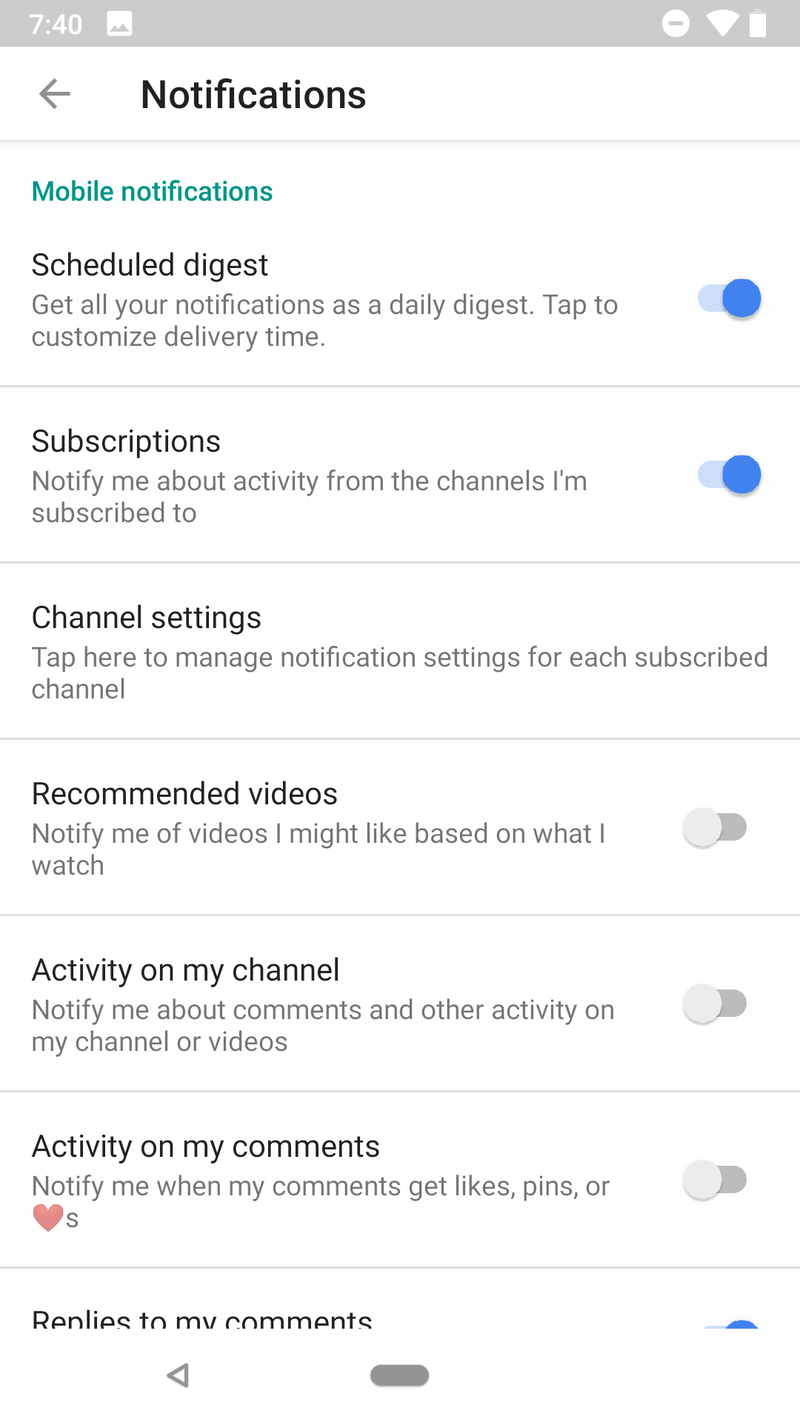This is a detailed screenshot of the notification settings page from a mobile app on someone's phone. 

At the top, there's a slim, rectangular gray bar displaying "7:40" on the left side, with a small icon next to it. To the right of that, you see the Wi-Fi signal indicator, battery status, and a circular symbol.

Directly below, the page is headed with "Notifications" followed by a left-pointing arrow icon. Below, it displays the "Mobile notifications" section, featuring several settings divided under subheadings.

First is "Scheduled Digest," with a description beneath it stating, "Get all your notifications as a daily digest. Tap to customize delivery time." There's a toggle switch next to this option, which is currently switched on.

Next, the "Subscriptions" section reads, "Notify me about activity from the channels I'm subscribed to," accompanied by another toggle switch.

Following that, "Channel Settings" prompts, "Tap here to manage notification settings for each subscribed channel."

Then, there's the "Recommended Videos" section, stating, "Notify me of videos I might like based on what I watch."

Below, the "Activity on My Channel" section mentions, "Notify me about comments and other activity on my channel or views videos."

Finally, "Activity on My Comments" reads, "Notify me when my comments get likes, pins, or hearts," with most switches below these headings toggled off, except for the first two which are toggled on in blue. Additionally, there is a partially visible button labeled "Replies to my comments" that is turned on but not fully shown in the screenshot.